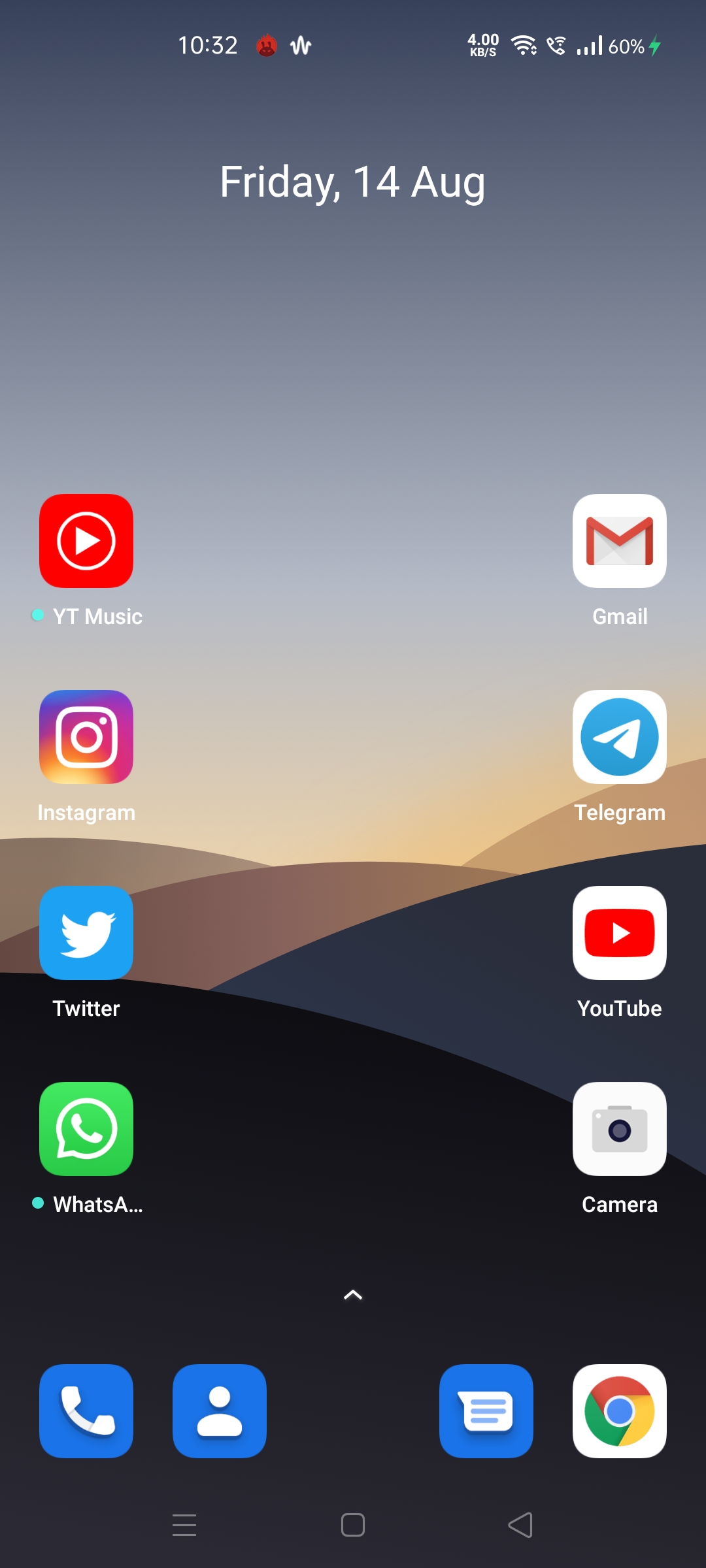The image depicted is in portrait mode with a background that starts off as a solid gray at the top and transitions into an abstract pattern featuring hills of brown, dark brown, gray, and black towards the bottom. At the top-center of the screen, it reads "10:32," while the top-right corner displays a battery icon indicating "60%" with a green lightning symbol signifying charging. Below this, the text "Friday, 14 August" is prominently displayed.

The screen is populated with a grid of app icons. On the left side, the first row includes "YT Music" accompanied by a little green dot, and on the right side, "Gmail." The second row features "Instagram" on the left and "Telegram" on the right. The third row shows "Twitter" on the left and "YouTube" on the right with its red and white play button icon. The fourth row bears "WhatsApp," marked with a green button circled next to it, and "Camera" on the right. 

At the bottom of the screen are additional icons placed in a row, including the phone app, a person icon, the messaging app, and Google Chrome. Each app name is paired with its corresponding icon, such as the Twitter bird, Instagram's rainbow gradient camera, and WhatsApp's green speech bubble.